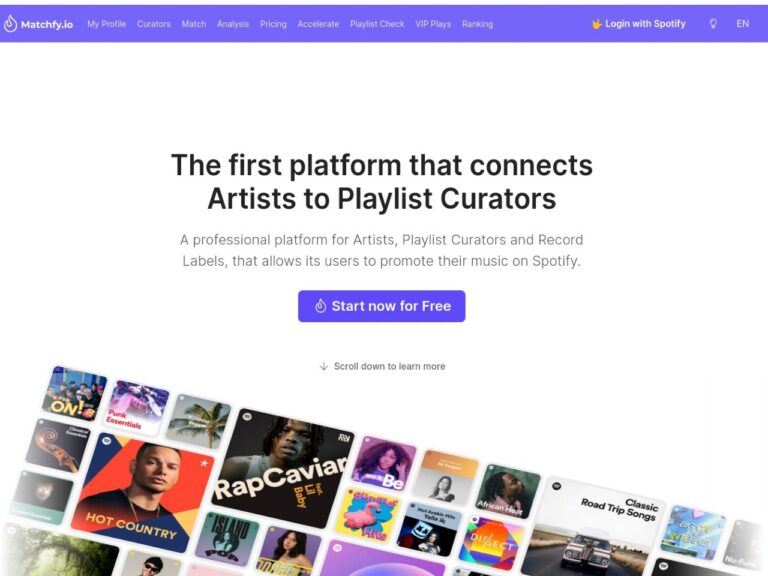### Detailed Caption for the Image

This image is a landscape-oriented screenshot likely taken from a laptop. 

### Upper Section
- **Header Strip**: The top section features a purple background strip, with text that is notably difficult to read due to its light font color.
  
- **Top Left Corner**:
  - **Logo**: The logo "MATCHFY.IO" is prominently displayed.
  - **Category Headings**: A series of headings are displayed, including "My Profile," "Curators," "Match Analysis," "Pricing," "Accelerate," "Playlist Check," "VIP Plays," and "Ranking."

- **Top Right Corner**:
  - **Login Section**: There's a noticeable yellow mark followed by the text "Log in with Spotify."
  - **Language Option**: An icon is displayed next to the language selection "EN English."

### Main Content Area
- **Background**: The main section has a white background.
  
- **Central Text**:
  - **Main Heading**: "The first platform that connects artists to playlist curators."
  - **Subheading**: "A professional platform for artists, playlist curators, and record labels that allows its users to promote their music on Spotify."
  
- **Call-to-Action Button**: A prominent purple button labeled "Start Now for Free."
  
- **Instructional Text**: Below the button, there's a line of text that reads "Scroll down to learn more."

### Lower Section
- **Large Image**: Occupying the lower section of the screenshot is a large composite image showcasing different selections and album covers on Spotify.
  - **Featured Categories**: Categories such as "Hot Country," "RAP Caviar," and "Classic Road Trip Songs" are visible.
  - **Album Covers**: Various album covers, presumably from different artists, are displayed in a collage-like format, depicting a snapshot of Spotify's diverse offerings.

Overall, the screenshot appears to be from a music-related platform, MATCHFY.IO, designed to connect artists with playlist curators, displayed in a clean, professional layout with straightforward navigation and call-to-action prompts.